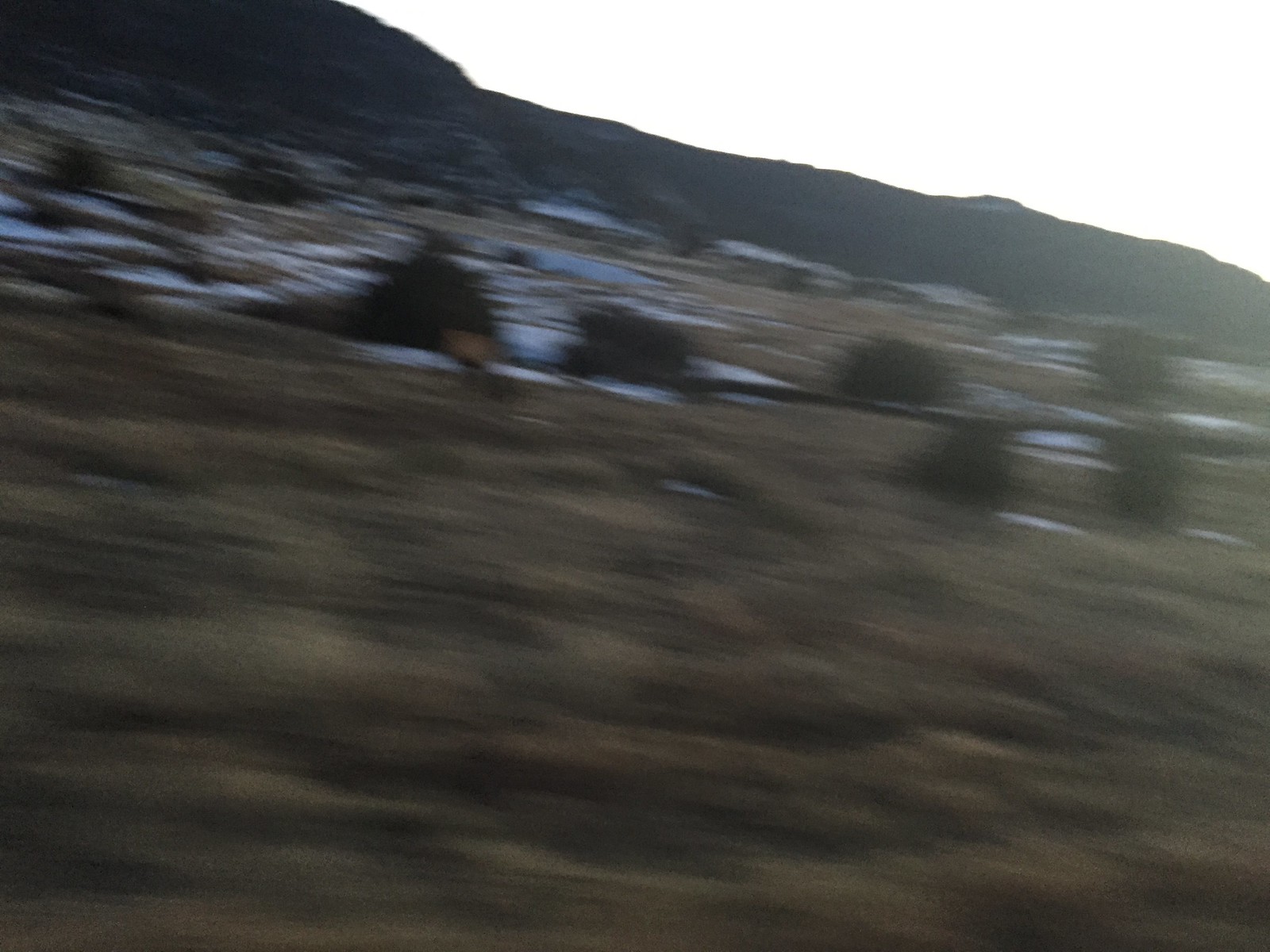This is a blurry, out-of-focus photograph, likely taken from a moving car. The landscape features a prominent mountain in the background with patches of melting snow scattered along its base. In front of the mountain, there's a field with a mix of light yellow dead grass and darker green bushes. Toward the foreground, there's some sand and more dead grass, adding to the arid appearance. The sky appears to be pure white, possibly due to overexposure. The overall scene feels desolate with hints of greenery, hinting at a transition from winter to spring. The blurriness suggests the photograph was taken quickly, capturing the motion and haste of the photographer.